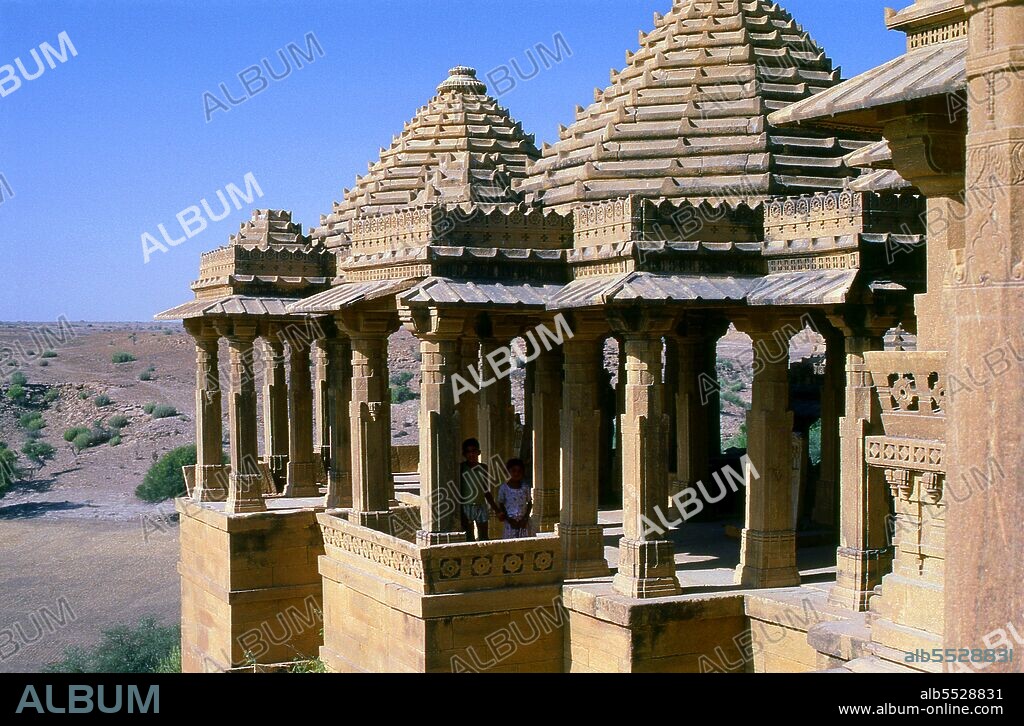This is a stock photograph of an ancient temple, possibly Tibetan or Thai, located in the middle of a dry desert landscape dotted with green bushes. The temple structures appear to be made of tan stone and feature intricately carved, tiered roofs, giving them a distinctive, pointed appearance. The base of these temple towers is supported by elaborately decorated pillars, and there are areas that seem designed to provide shade or channel water. In the foreground, two children stand beneath the central structure, highlighting the scale of these towering edifices. The image is heavily watermarked with the word "album" repeated multiple times, and at the bottom of the photo, there is a black line with the text "album" on the bottom left and a website address, www.album-online.com, along with a serial number, ALB5528831, on the bottom right. The overall color palette of the image includes dull tones of brown, beige, and gray, contrasted by the blue sky in the background.